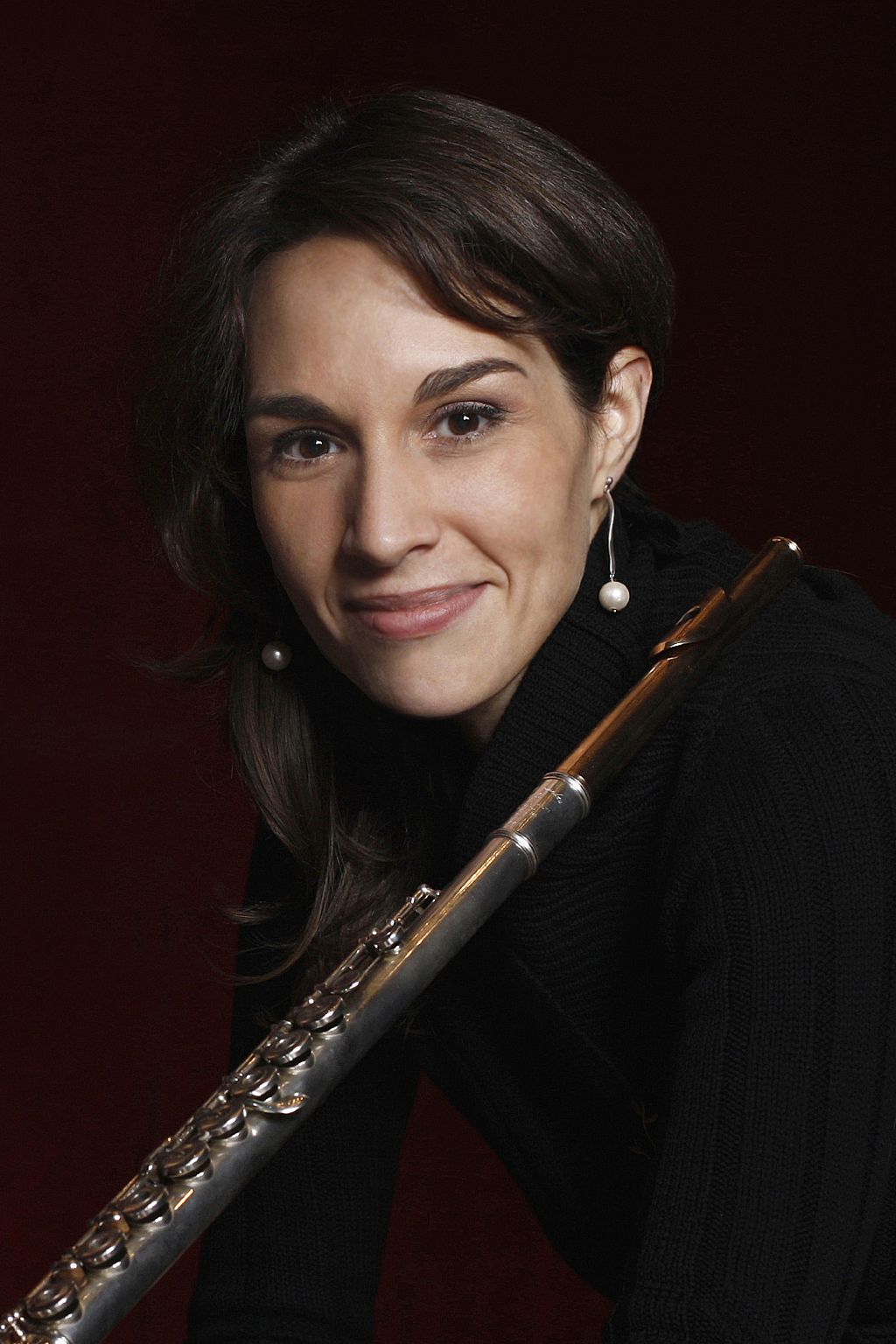The photograph captures a female musician in her mid-to-late 30s with an instrument, likely a silver flute, resting over her left shoulder. She has dark brown, shoulder-length hair, neatly groomed with the left side tucked behind her ear, while the right side cascades over her face. Her olive-toned skin is complemented by dark, expressive eyes and thick, beautifully manicured eyebrows. She sports pearl earrings that dangle elegantly, aligning with her sophisticated yet understated look. Her lips are a pale red, forming a closed-mouth smile that exudes a confident charm. She is dressed in a dark turtleneck, leaning slightly forward with her torso and above visible. The background is a dark, rich color, possibly magenta or black, providing a striking contrast that highlights her facial features and the flute. The image radiates a professional yet alluring vibe, suitable for use in promotional materials like a website or brochure for a musician.